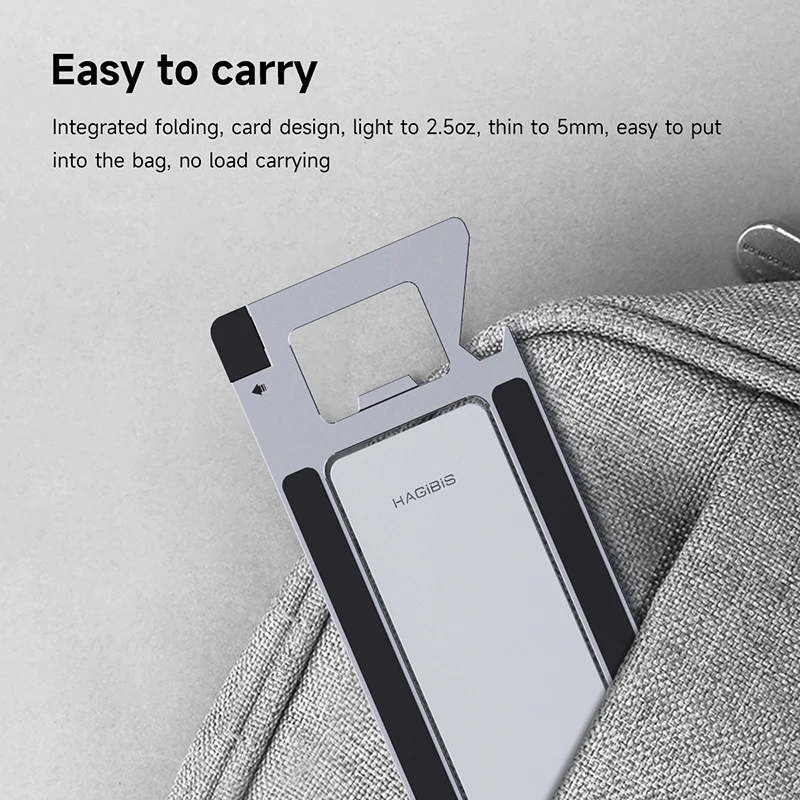The image is an advertisement for a phone accessory branded "Hagibis," designed as a versatile, easy-to-carry holder or stand. It prominently features black text at the top, stating key attributes: "Easy to Carry, Integrated Folding, Card Design, Light to 2.5 Ounces, Thin to 5 Millimeters, Easy to Put into the Bag, No Load Carrying." The accessory itself is sleek and lightweight, weighing just 2.5 ounces and measuring only 5 millimeters in thickness, making it exceptionally portable. It has a distinctive square hole at the top with a narrow opening, indicating multifunctional use, potentially as a bottle opener, can opener, or letter opener. The device is integrated into a pocket of a stylish tweed-like gray and white bag, which rests on a gray surface, emphasizing its compatibility with everyday carry items. Despite not having visibility into the bag's interior threading condition, the overall presentation underscores both convenience and practicality, ideal for on-the-go usage.